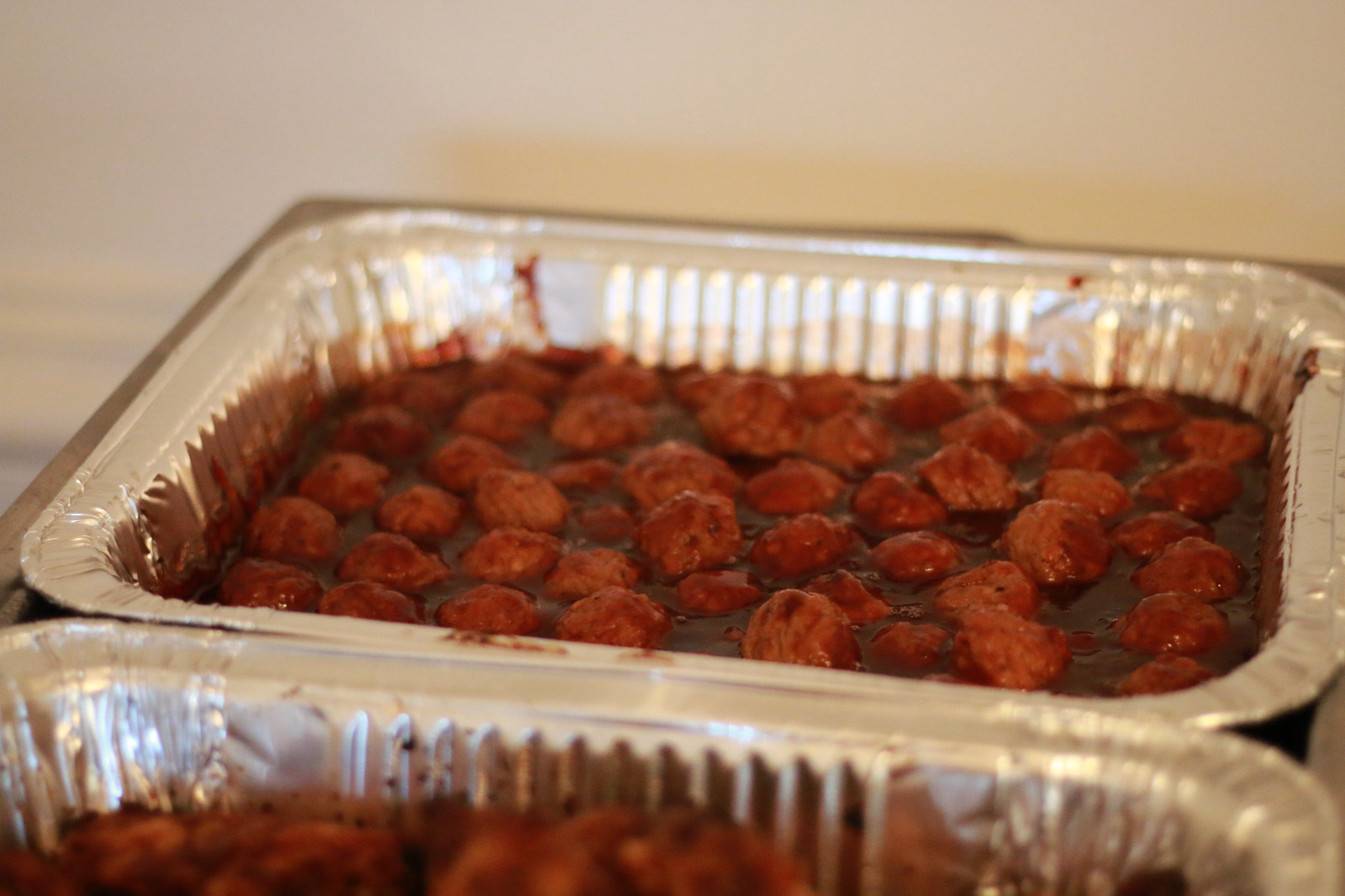This is an up-close shot of two rectangular metal baking pans, commonly used for takeout. The scene is simple, with the pans resting on a white background and no visible table setting. The pan in the foreground is slightly out of focus, revealing only a vague impression of its contents, which appear to be similar in style and color to the second pan. The second pan, which is in clear focus, is filled with approximately 50 small, cooked meatballs, possibly turkey due to their lighter color compared to beef. They are covered in a browned red sauce that clings to the edges of the pan, suggesting it could be either barbecue or tomato-based. The meatballs are arranged loosely in a pattern but without perfect uniformity. The second pan is not fully filled and appears about halfway full, contributing to the image’s casual, homely feel.